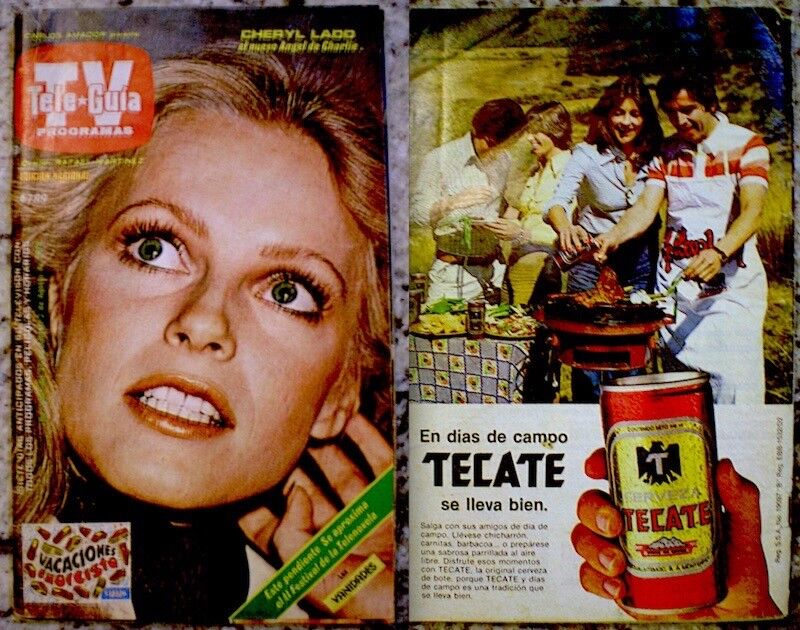This detailed photograph showcases an opened Spanish version of a TV guide magazine. The left side features the front cover with a close-up of Cheryl Ladd's head and shoulders, showing her looking up and to the right. The title "Telegia" is displayed in a red square in the upper left corner, and "Angel de Charlie" appears in yellow text, indicating her role in Charlie's Angels. In the upper corner, "Programas" is also visible, emphasizing its TV guide content. On the right side of the photo, the back cover is prominently shown, presenting a vibrant advertisement for Tecate Beer. The ad features a hand holding a recognizable red and gold Tecate can, along with the text "En Días de Campo, Tecate se lleva bien." The scene above the text depicts two couples enjoying a barbecue outdoors; one couple is actively grilling while the other couple stands beside a table set with food, surrounded by trees, with the woman smiling warmly at the man. The overall aesthetic evokes a nostalgic 1970s feel.